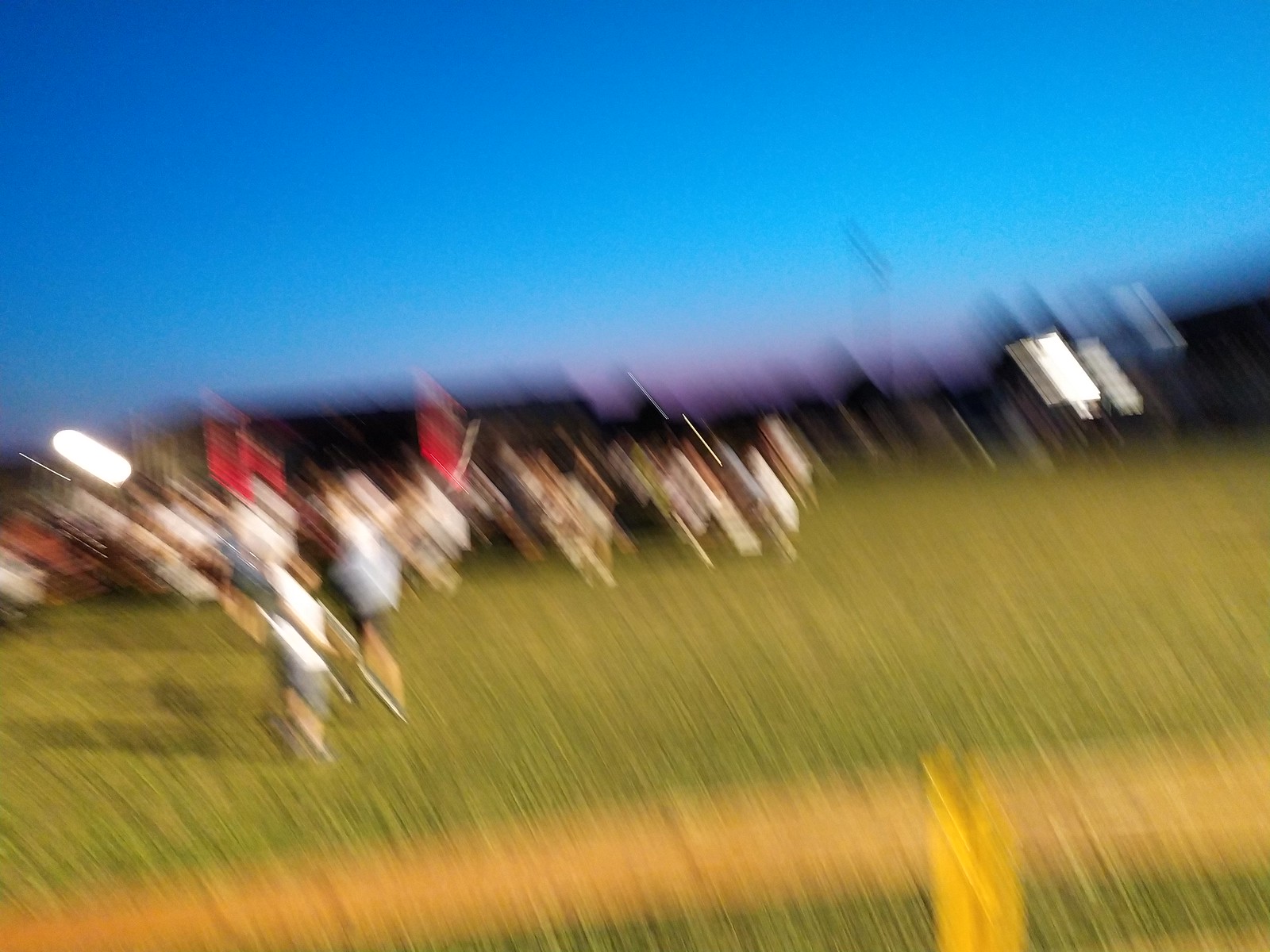The photograph taken around dusk captures a blurry outdoor scene with a deep blue sky dominating the upper half and a green field below. The blue sky has a medium hue indicative of evening time. The green area, presumed to be grass, is intersected by a dirt road or path that runs horizontally. In the bottom right, a yellow marker or line suggests it could be a football field. The photo’s central focus is a blurred crowd, possibly children, with some appearing to wave objects amidst a vertical blur that distorts their forms into indistinct shapes and colors. Amid this blur, some viewers interpret the presence of red and silver hues, reminiscent of Roman warriors or armor. An illuminated structure, possibly a house, brings additional light to the scene from the right side.